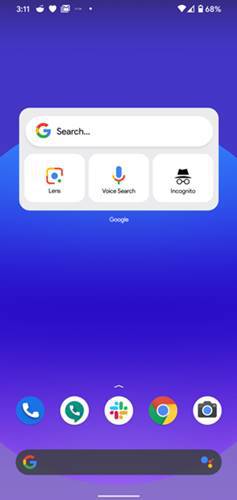The image is a screenshot of a smartphone home screen. The time displayed in the upper left-hand corner is 3:11. To the right of the time, there are three icons: the first icon is indiscernible, the second icon is a heart, and the third icon is also indiscernible.

On the upper right-hand side, the Wi-Fi signal indicator is shown in white. Next to it is the cellular signal strength indicator, depicted as a triangle. The battery life is displayed at 68%.

Below the status bar, there is a Google search bar featuring the multi-colored Google "G" logo and the word "search." Directly beneath this search bar are three buttons: "Lens" with the Google Lens logo, "Voice Search" with a microphone icon, and "Incognito" with a black and white icon of a hat and glasses.

Further down, a row of app icons is visible. From left to right, these include: the Phone app, the WhatsApp app, another indiscernible app with multi-colored dots, the Chrome app, and the Camera app. All icons are circular.

At the bottom of the screen, there is a second Google search bar, this time in black with the same multi-colored Google "G" logo.